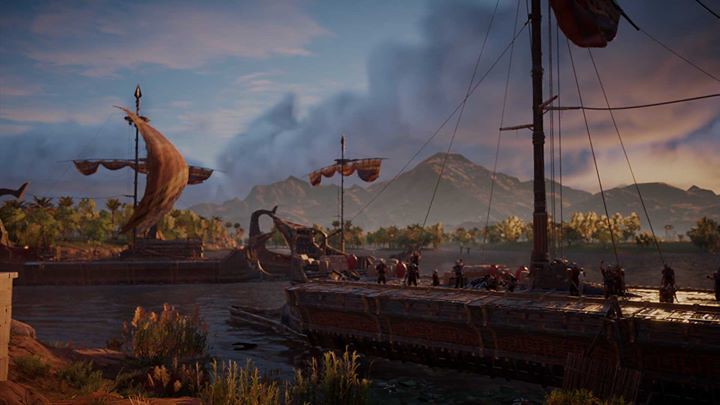This painting depicts a serene body of water featuring three majestic, old-fashioned sailing ships with light brown sails. In the immediate foreground, small grasses populate a gentle bank leading down to the water's edge. The ships, rendered in shades of brown, dominate the scene with their sizeable presence, yet the figures of the men aboard appear diminutive by comparison. Beyond the tranquil waters, a hill adorned with a cluster of slender palm trees gives way to imposing mountains. These mountains, draped with a rich tapestry of trees, ascend towards the sky which transitions from a clear light blue overhead to grayish clouds that hover above the mountainous horizon. The water below reflects a brownish hue, mirroring the earthy tones of the ships that traverse it.